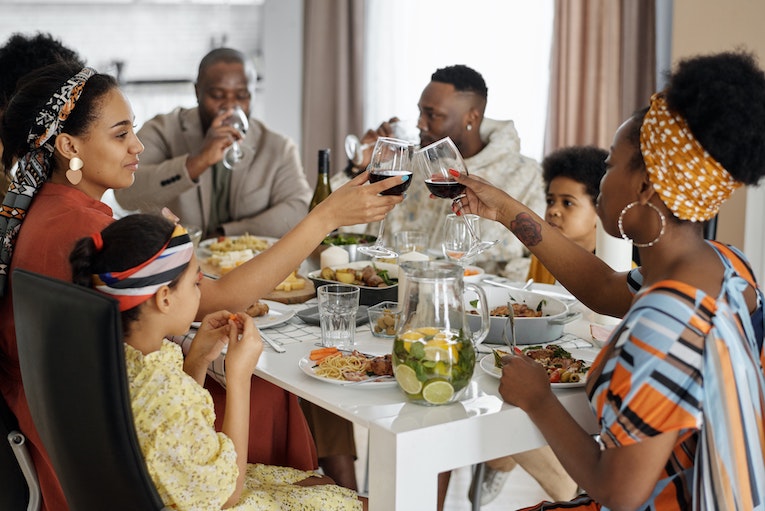In this detailed photo, an African-American family is gathered for a joyous dinner around a white wooden kitchen table adorned with black and silver chairs. The table is laden with an inviting spread of spaghetti, carrots, chicken, and potatoes. A clear glass pitcher filled with lemon and lime-infused water sits prominently among the dishes. Seated on one side are two men enjoying glasses of wine, while opposite them, two women in vibrant orange, yellow, and blue dresses, with coordinating headscarves, toast each other with their wine glasses, beaming fond smiles. Completing the scene, a young boy and girl, the latter wearing a striped headband and yellow dress, also sit around the table, fostering a sense of warmth and togetherness. This lively and colorful depiction encapsulates the spirited essence of a family gathering, richly detailed and harmoniously bonded.